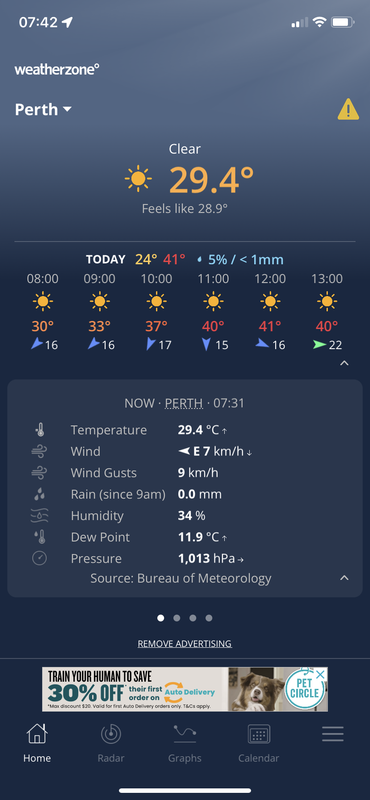**Detailed Caption:**

A screenshot of a weather application interface with a multi-hued blue gradient background, which transitions from a lighter shade at the top to a darker shade at the bottom. The screen displays the time "7:42" with an error notification indicated by an upward-pointing arrow. Only two signal bars are visible, yet the battery shows a solid performance at approximately 80% charge. 

Displayed prominently in the center, the app title "Weather Zone" is written in lowercase white letters, followed by the location "Perth," presumably Perth, Australia. To the right is a drop-down menu icon and a triangle with an exclamation mark, signaling a weather warning.

The current weather status reads "Clear" in white letters, accompanied by an orange-yellow icon symbolizing sunshine and the temperature listed as 29.4 degrees. The "feels like" temperature of 28.9 degrees is shown in smaller gray text, although the scale (Celsius or Fahrenheit) is unspecified. It also notes that today's low is 24 degrees, with a high of 41 degrees, and indicates a less than 5% chance of rain.

The seven-day forecast runs horizontally across the screen, showing daily high temperatures of 30, 31, 37, 40, 41, and 40 degrees. Below this, there is additional detailed information about Perth, featuring various clickable elements for further weather details and updates. The interface is comprehensive, providing a thorough overview of the current weather conditions and future forecasts.